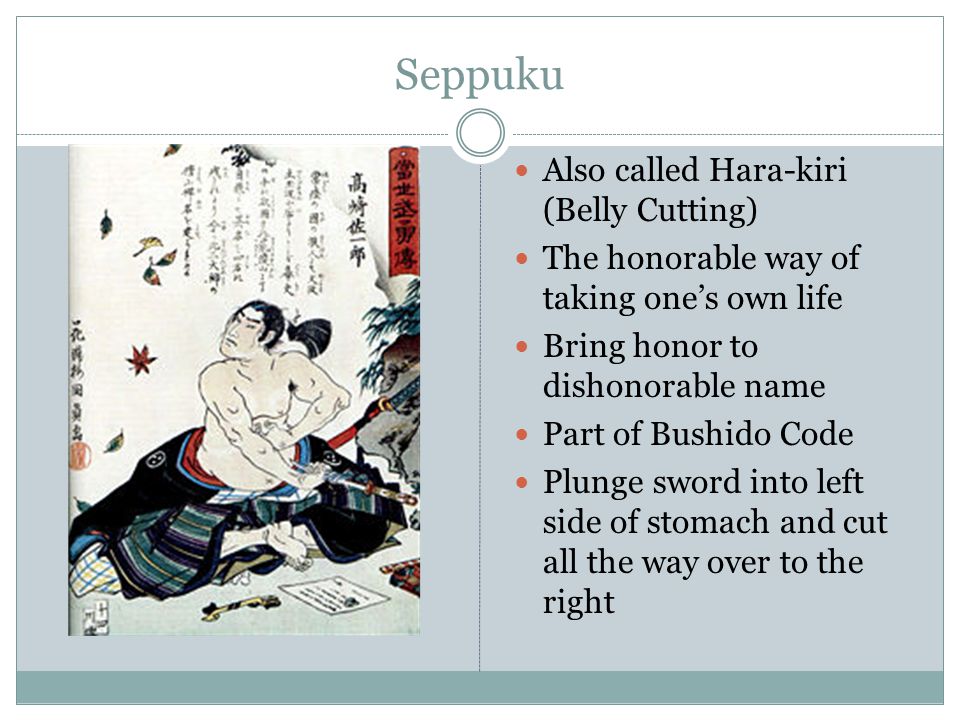The digital presentation slide features a detailed overview of the Japanese ritual of seppuku, also known as harakiri or "belly-cutting." The slide is on a mostly light gray background with a dark teal border at the bottom. At the top, in light blue lettering, is the title "Seppuku." The slide is divided into two main sections: on the left side, there is an illustration of a somber-looking samurai or Japanese man performing seppuku, depicted without a shirt and in traditional attire, with long black hair tied back. He is shown plunging a sword into his stomach while surrounded by papers and supplies. The background of the illustration is white. 

On the right side, within a separate box, there are several bullet points in red detailing the concept of seppuku. The bullet points are as follows:
1. Also called harakiri (belly-cutting).
2. The honorable way of taking one's own life.
3. Bring honor to a dishonorable name.
4. Part of the Bushido code.
5. Plunge sword into the left side of the stomach and cut all the way over to the right.

The content provides a comprehensive understanding of the ritual, emphasizing the method and cultural significance behind it.